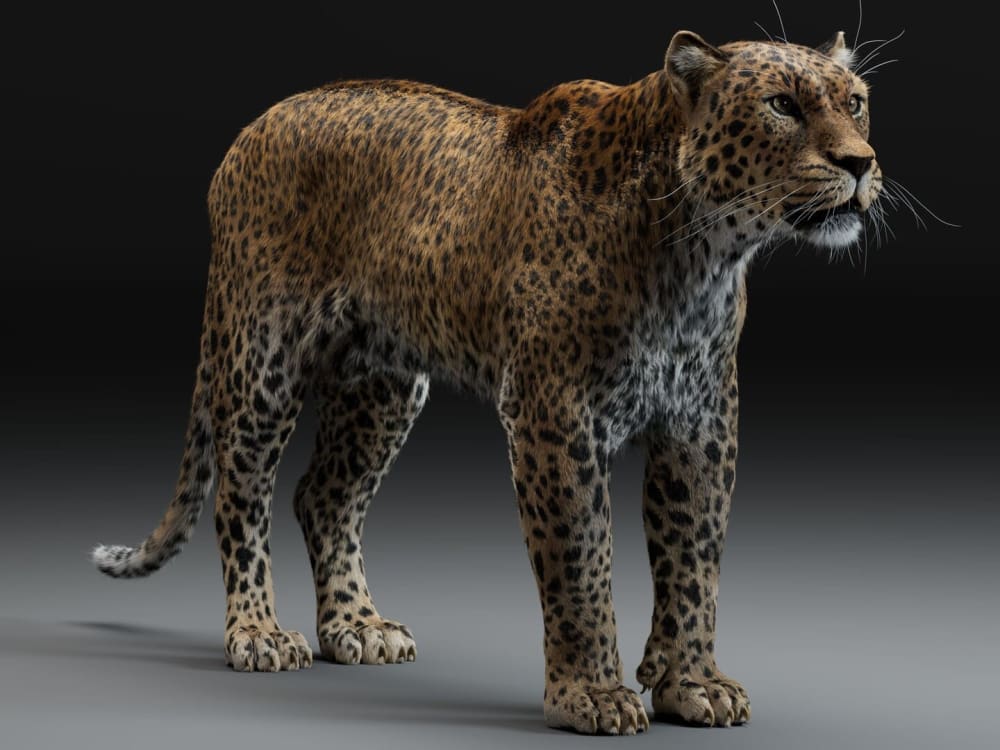This image is a digitally created painting of a large wild cat, likely a cheetah or leopard. The animal stands on a gray floor that fades seamlessly into a black background, giving the impression of a moody, shadowy environment. The rendering is so detailed and realistic that it almost appears as though it could be a taxidermy specimen. The cat's body displays a mesmerizing pattern of black and brown spots on a golden yellow to orange coat, with additional black and white spots adorning its legs and chest. Its face, captured in near profile but fully visible, is distinguished by a set of prominent whiskers emanating from both its mouth and above its eyes. The cheetah stands with a looped tail behind it, exuding a lifelike yet almost eerie stillness. The overall scene lacks other objects or text, focusing entirely on the serene yet powerful presence of the cat.